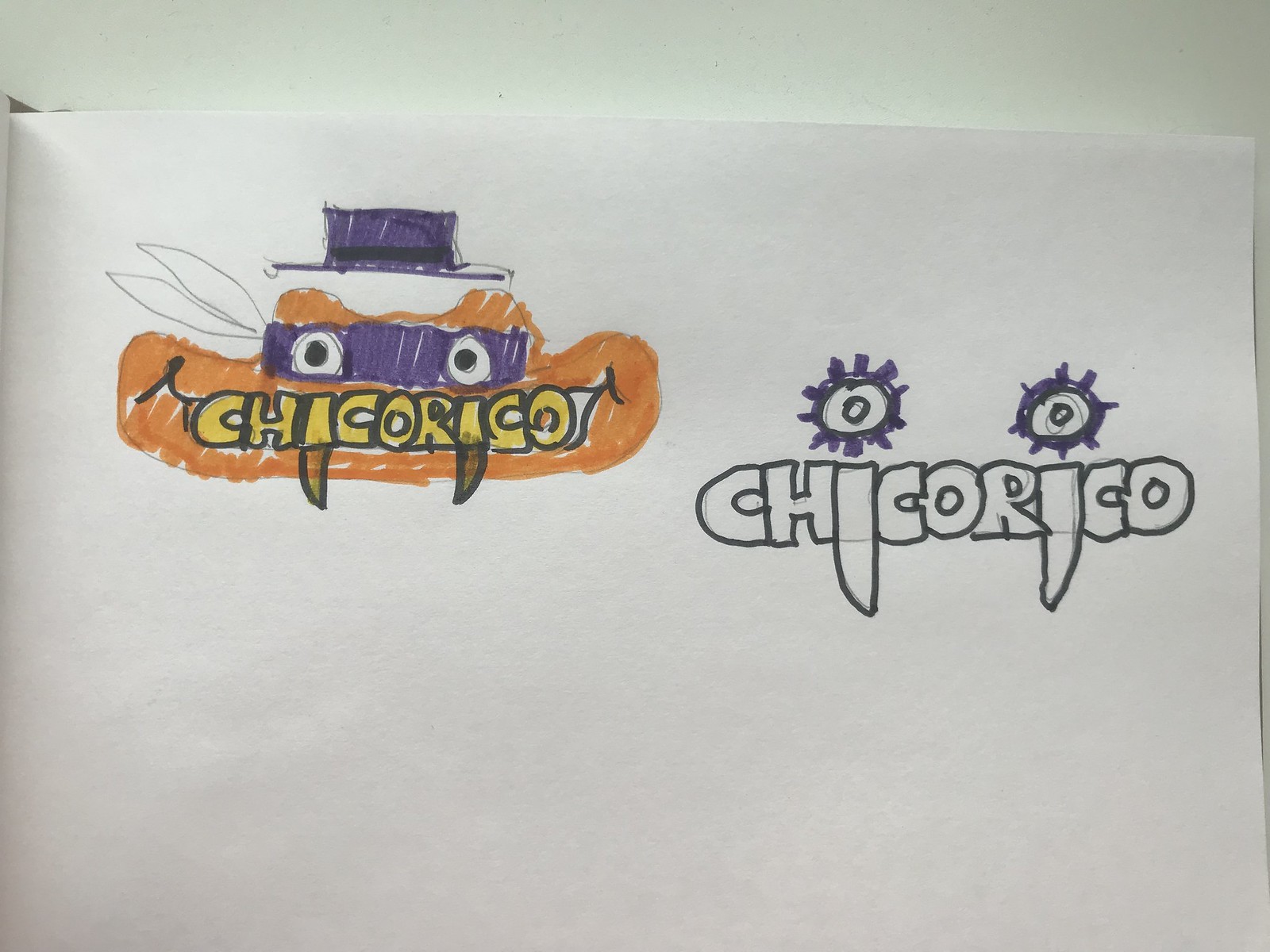The image is of a piece of white construction paper featuring a hand-drawn character resembling a bandit. On the left side, there's the logo "Chico Rico" written in black marker, with the letters C-H-I-C-O-R-I-C-O. The character has an orange face resembling a wide, big mouth duck and is detailed with a purple hat that has a black ring around it. The eyes of the character are white with black pupils and feature purple eyelashes, giving the appearance of a mask. The mouth is wide and long, with prominent fangs. The same character appears on the right side of the paper, but without any colors filled in, just the pencil outlines. The name "Chico Rico" reappears in black and white letters with eyes formed within the letters, featuring the same fang shape. The overall look is that of an orange bandit face with a purple mask and hat, emphasizing the detailed, colored version on the left and the outlined, colorless version on the right.